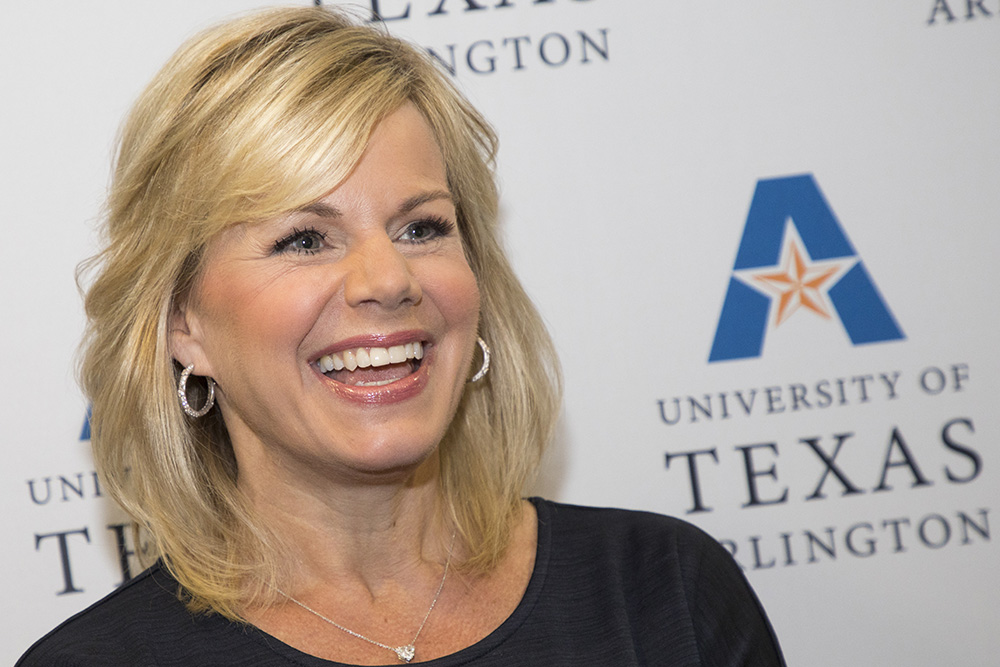In this image, a woman stands indoors, her position slightly off-center while facing right, exuding a vibrant and joyous aura with an open-mouth smile. Her styled blonde hair complements the silver hoop earrings adorned with tiny gemstones and a necklace featuring gemstones and a small locket. She is dressed in a black shirt, further highlighting her accessories. The background showcases a white wall with the repeated text "University of Texas Arlington" and the institution's logo—a stylized blue 'A' with a white and gold star. The overall color palette of the image includes black, white, blue, orange, pink, tan, and yellow, evoking a colorful yet cohesive scene. The setting suggests an indoor college environment aimed at capturing genuine and happy moments.